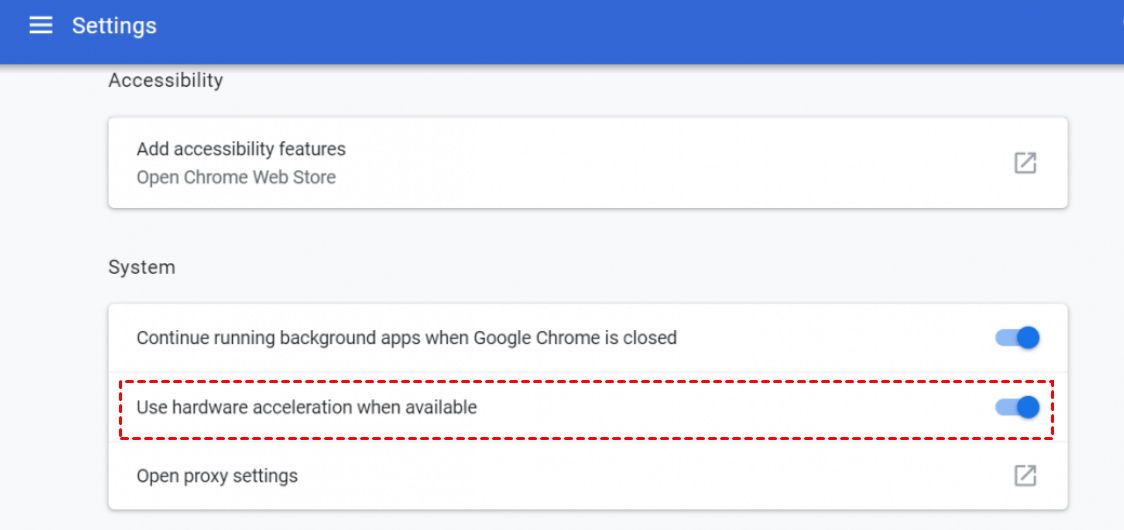On a gray background, a blue header features a hamburger icon and settings icon in white. Below, a white rectangle contains the title "App Accessibility Features" and a prompt to "Open Chrome Web Store." To the right, there's an icon of a square with a diagonal arrow pointing up and to the right, labeled "System." 

Another white rectangle is divided into three sections:

1. The first section displays "Continue running background apps when Google Chrome is closed" with the toggle bar turned on, followed by "Use hardware acceleration when available," again with the toggle bar turned on.
2. The second section is outlined by a dashed red line forming a rectangle.
3. The third section offers "Open proxy settings" accompanied by an icon of a square with a diagonal arrow pointing up and to the right.

The overall layout highlights various accessibility and system settings in Google Chrome, with key options emphasized for user interaction.